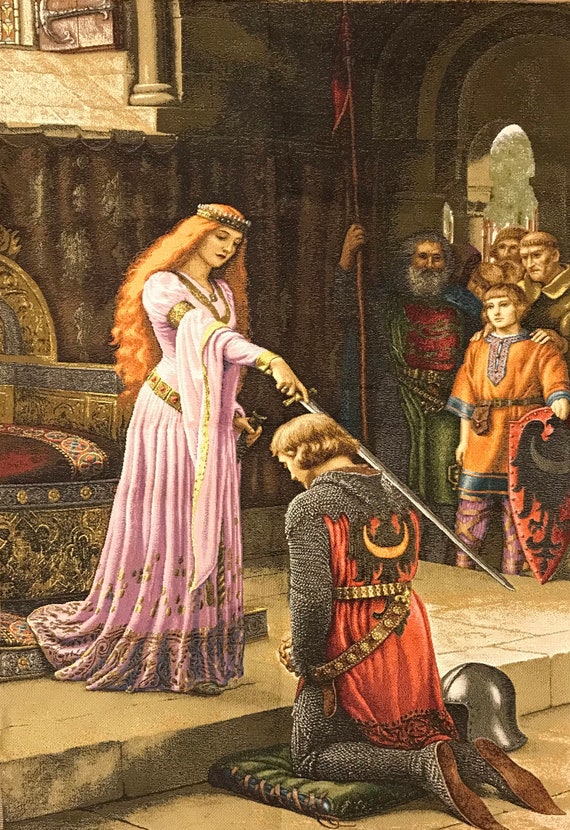In this detailed, portrait-oriented painting, a medieval lady is depicted knighting a man in chain mail. She stands on a raised dais with an intricate throne behind her, illuminated by sunlight streaming through a window above. The lady, serious in demeanor, has very long curly red hair adorned with a metallic headband or crown. She wears a light purple lilac dress with gold jewelry and highlights as she holds a sword, placing it on the knight's right shoulder. The knight, kneeling on a green cushion, is dressed in dark gray chain mail under a red tunic, and his helmet is placed beside him. He sports pointy leather shoes and a gold belt. Several observers stand near an archway in the background, including a monk with tonsured hair, an older knight holding a red flag on a stick, a squire in an orange cloak holding a red shield, and another indistinct bearded man. The scene is rich with intricate details, capturing a solemn and ceremonious moment in a fairy-tale-like setting.